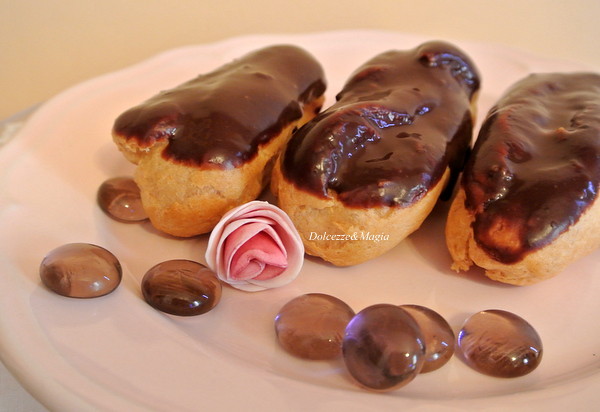This detailed close-up photograph showcases a round, white plate adorned with three oblong chocolate éclairs, each topped with a glossy chocolate icing. These tan pastries are aligned diagonally, stretching across the plate on a beige surface. In addition to the pastries, the plate features a small pink rose, nestled between two of the éclairs, and a scattering of seven clear, flat glass stones resembling stones from a Mancala game. There is superimposed white text over the middle éclair that reads "dolcez e magia." The ambiance hints at a fusion of French and possibly Asian influences, likely suggesting a Vietnamese bakery or similar establishment.